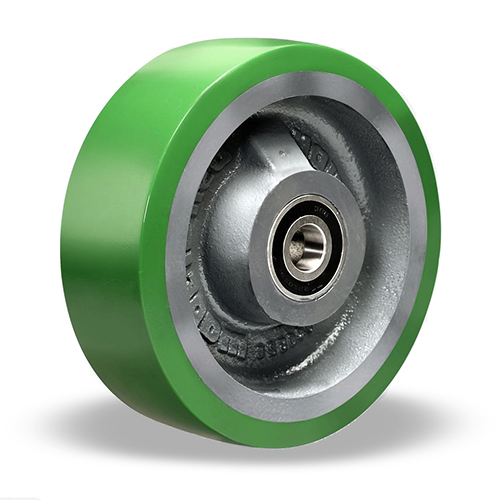The image depicts a 3D object that resembles a wheel or gear, possibly for a skateboard or a lock mechanism. The outer rim is pea green, while the inner sections are composed of silver metal. There are letters or text etched into the metal around the middle border, although they are difficult to decipher, with one notable letter being "W." The center of the object features a black o-ring or bearing, enhancing its mechanical appearance. The wheel-like object is shiny and detailed, with visible grooves and circular decorations. The background is plain white, providing no additional context about the object's use.